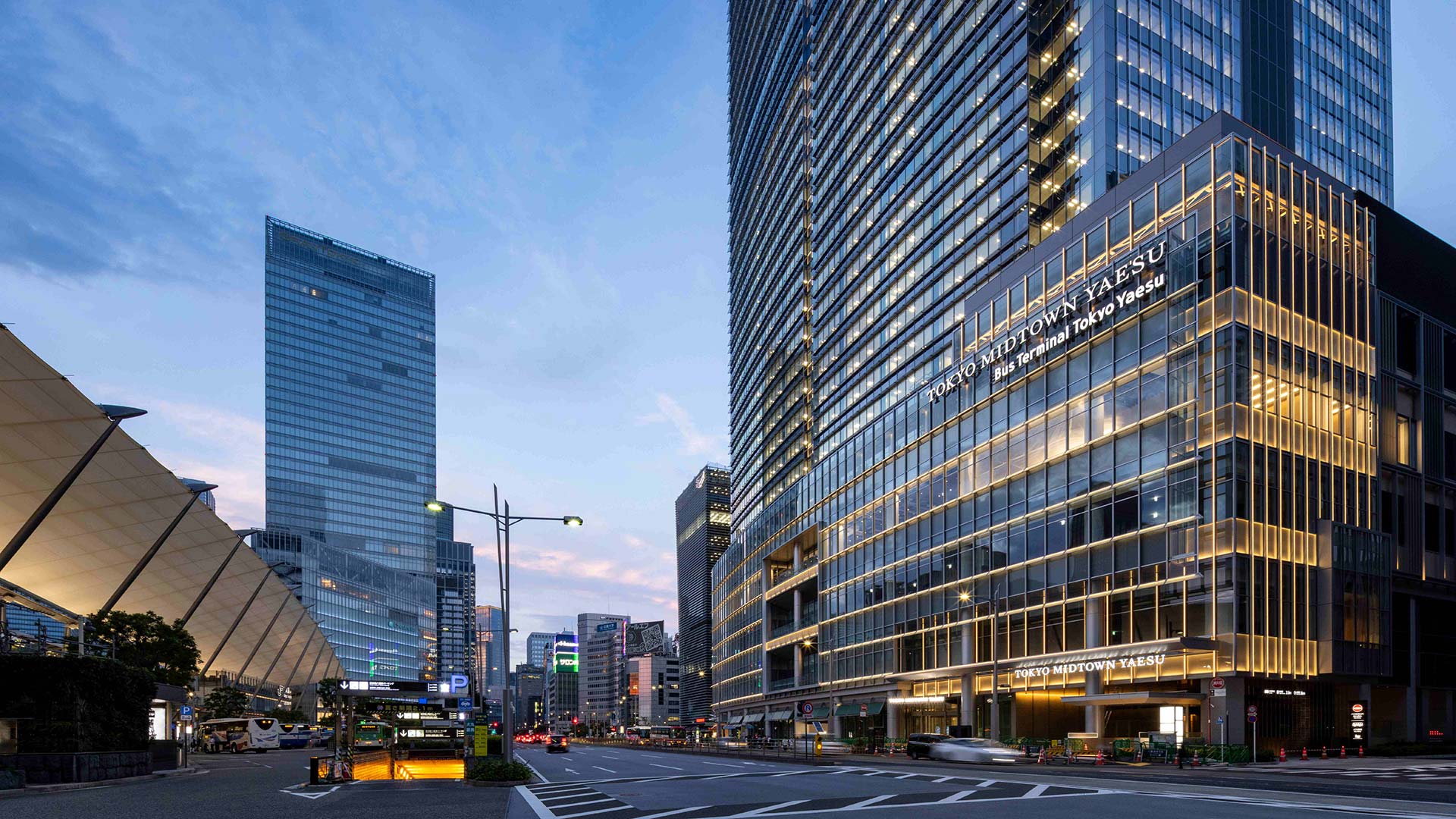This is a photographic image capturing a city street at night, likely the early evening or dusk, in Tokyo, Japan. The photo is taken from the perspective of someone standing on the street, looking down towards the intersection. 

In the foreground, on the bottom left corner, there is a visible fabric tent held up by numerous poles, set on a backward incline. Adjacent to this is a sidewalk that leads to an entryway to a subway station, accompanied by several potted plants. A prominent double-decker bus accentuates the city vibe.

The middle portion of the image features a four-lane grey street with white lane markings and light traffic moving away from the camera. 

On the left side in the background, there is a towering skyscraper made of glass and steel. Enhancing the urban atmosphere, a streetlight with two lamps and another street pole with dual lights can be seen.

On the bottom right corner stands a mid-level building, decorated with a sleek and polished black and gold facade. This modern building, presumably housing a restaurant and possibly apartments, has a sign that reads "Tokyo Midtown YAESU Bus Terminal," also repeated in smaller text beneath it. This text is a key identifier indicating the Tokyo Midtown YAESU area or bus terminal. 

There is a backdrop of clear blue sky with a few white clouds, hinting at the onset of early evening as the city transitions from day to night.